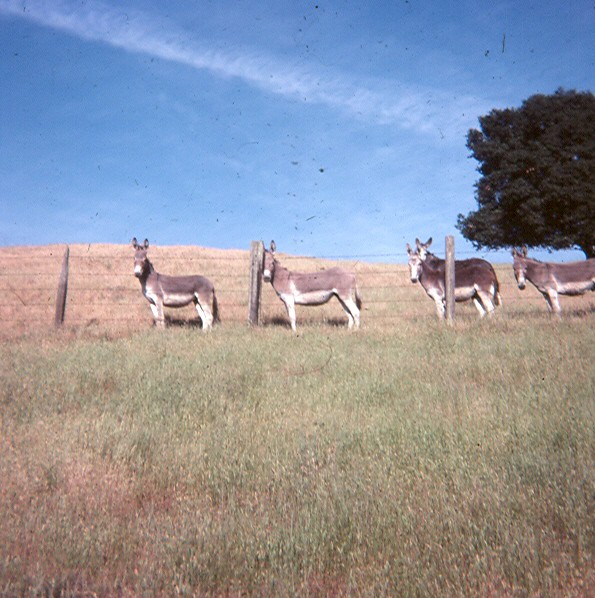The photograph captures a picturesque scene of five donkeys standing in a row on a hillside, just beyond a barbed wire fence made of four or five straight black wires strung between rustic wooden posts. The vibrant contrast between the lush green foreground of grass or weeds and the brown, drier pasture where the donkeys stand suggests they have been grazing. The donkeys, some of which have grayish-brown coats and others much darker gray, are all looking attentively towards the camera. The lineup is orderly, with the first three donkeys evenly spaced, the third standing parallel to another, and the fourth positioned closer to the rear of the one in front. Their coats feature white underbellies and legs, along with patches on their noses. The hillside ascends to a horizon punctuated by a large tree with a dense canopy of green leaves and a sky streaked with wispy clouds. Some black spots in the image could either be dirt or birds in the sky. Overall, the photo, taken from a slightly lower vantage point, gives a rustic feel with its mix of vibrant and muted natural tones, and a serene rural landscape bound by the wire fence, suggesting the donkeys are in a controlled pasture rather than roaming wild.